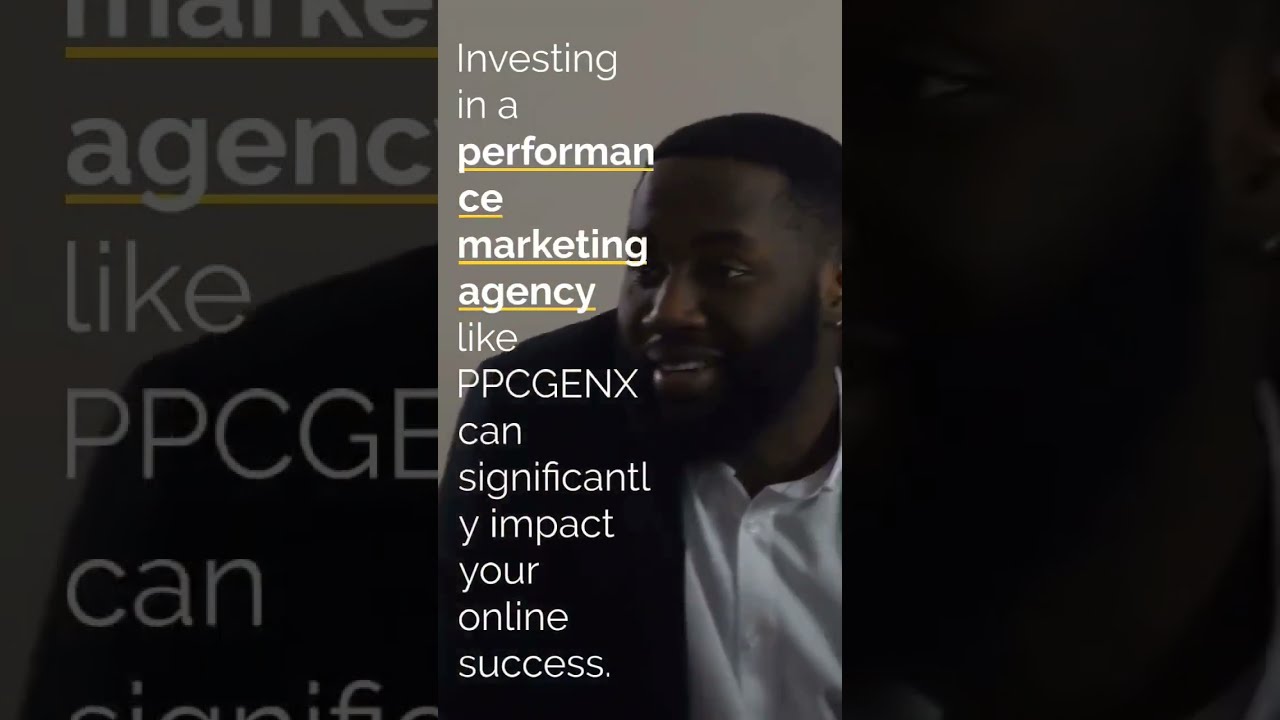The image is a horizontal rectangle, measuring approximately six inches wide and four inches tall, sectioned into three parts: left, center, and right. The center features a mid-chest-up photograph of an African American man with short black hair and a black beard and mustache. He faces forward with his head turned slightly to the left, appearing to speak with a smile. He wears a black jacket over a white button-down collared shirt, with the top button unbuttoned. 

From top to bottom, left-aligned white text occupies much of the image, reading: "Investing in a performance marketing agency like PPCGENX can significantly impact your online success." The words "performance" and "marketing agency" are emphasized with yellow underlines. The left section of the image enlarges and darkens the text "marketing agency like PPC," making it more prominent. Conversely, the right section is a close-up of the man's jacket, resulting mostly in a black area with little discernible detail. The overall appearance suggests the image is part of an advertisement or website for the performance marketing agency, PPCGENX.